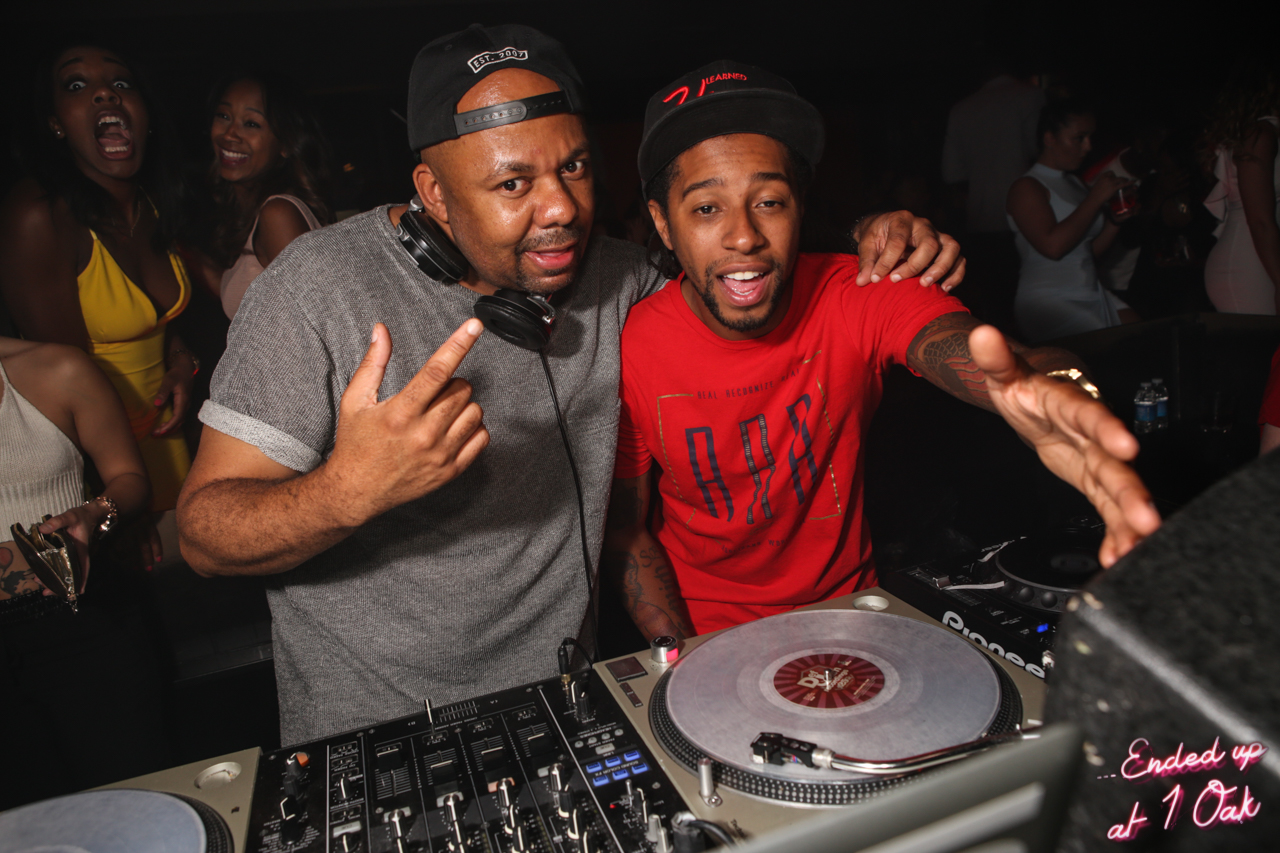This photograph captures an energetic moment inside a dimly lit nightclub, featuring two black men who appear to be DJs. The older man on the left is distinguished by his backward black hat and gray T-shirt with light gray borders. He wears a set of headphones and has his left arm draped over the shoulders of the younger man beside him. This younger man sports a forward-facing baseball cap with red lettering and a red T-shirt adorned with a design that includes three black stripes. Both stand in front of DJ equipment, including a turntable and a console. The older man is emphatically gesturing with his right hand, index finger pointing upward toward his ear. The background is filled with a lively crowd, including a woman in a low-cut yellow dress and another person in a white shirt, all enjoying the nightclub atmosphere. The bottom right corner of the image features pink lettering that reads "ended up at One Oak," possibly indicating the venue's name.